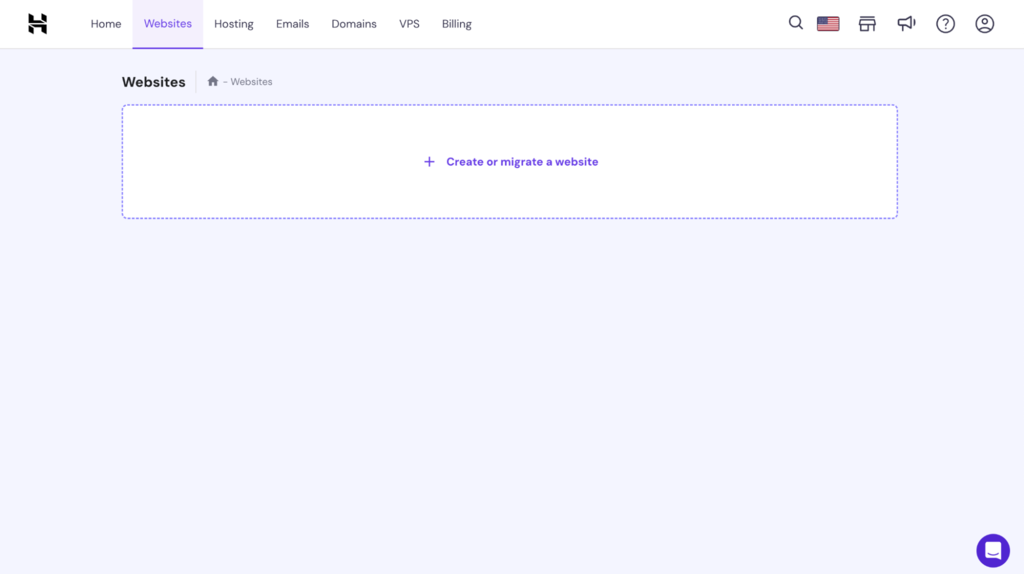This screenshot captures a user interface of a website creation platform, with its logo placed at the top left corner. The logo is somewhat ambiguous, resembling an 'H' symbol or potentially a stylized chair. At the top of the interface, a navigation menu is present, featuring options such as Home, Websites, Hosting, Emails, Domains, VPS, and Billing. The 'Websites' section is highlighted in purple text against a gray background, while the other options are displayed in black text on a white background.

On the right side of the top menu, several icons are aligned, including a search symbol, an American flag icon indicating language or region settings, a shopping cart, an announcement icon, a question mark for help or support, and a profile icon. 

Below the top menu, the main content area for the 'Websites' section is visible, set against a light blue/gray background. The word "Websites" is prominently displayed in bold, black letters. Next to it, a small house icon followed by the word "Websites" suggests a breadcrumb trail for easy navigation. A bordered rectangle area invites the user to either create or migrate a website, with the phrase "Create or Migrate a Website" highlighted in purple lettering inside this section.